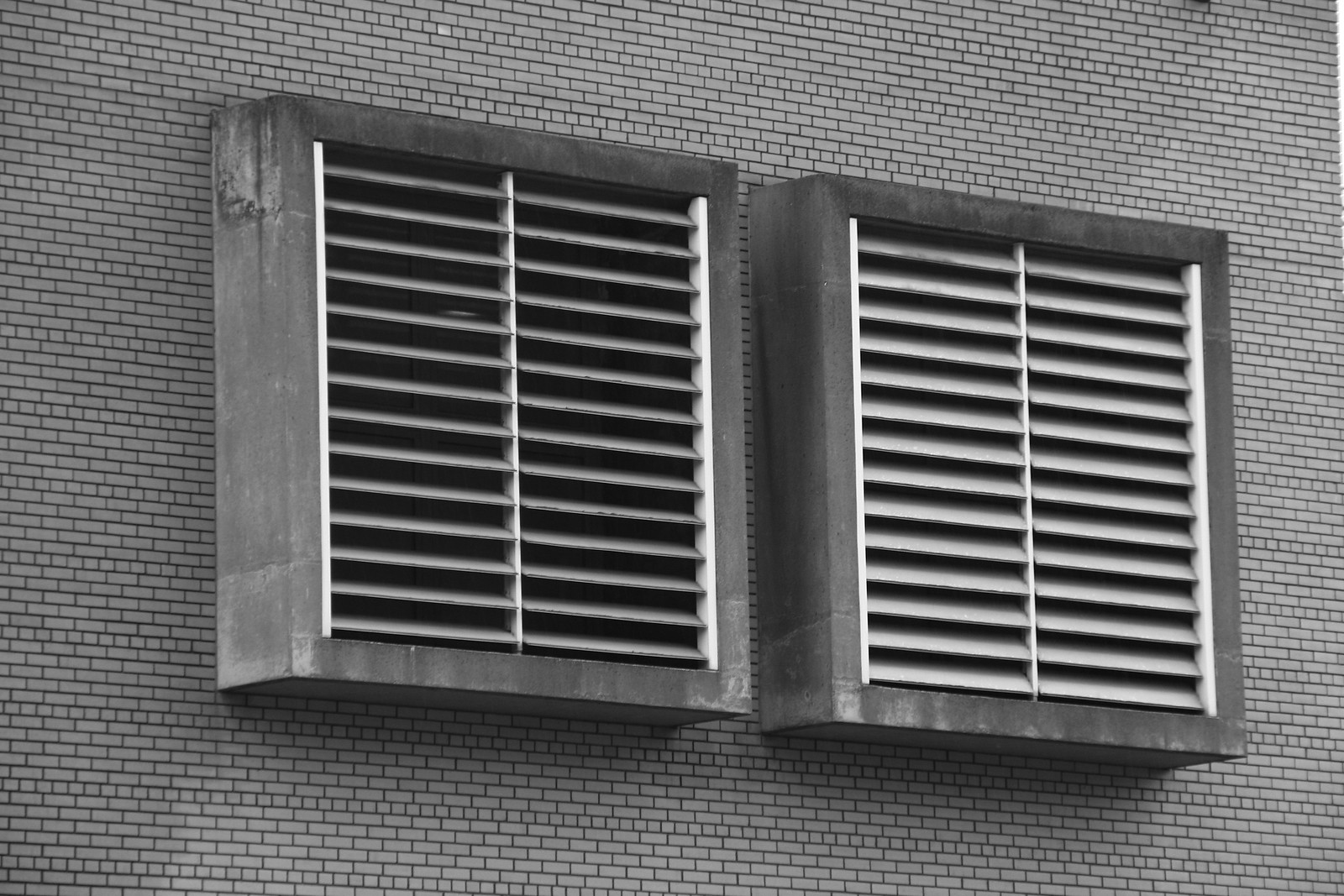This color photograph, taken outdoors, features a close-up view of a weathered brick building constructed from small, brownish-gray bricks. Prominently displayed in the center of the image are two large, white air duct vents. Despite being side by side, the vents are distinctly separated and are fronted by slanted metal grates, indicative of either intake or exhaust functionality. These ducts are encased in concrete, which shows signs of age with sections varying from grayish-black to nearly white, indicating weathering. The vents and ducts appear industrial and have a well-used look consistent throughout the image’s various shades of gray, black, and white.